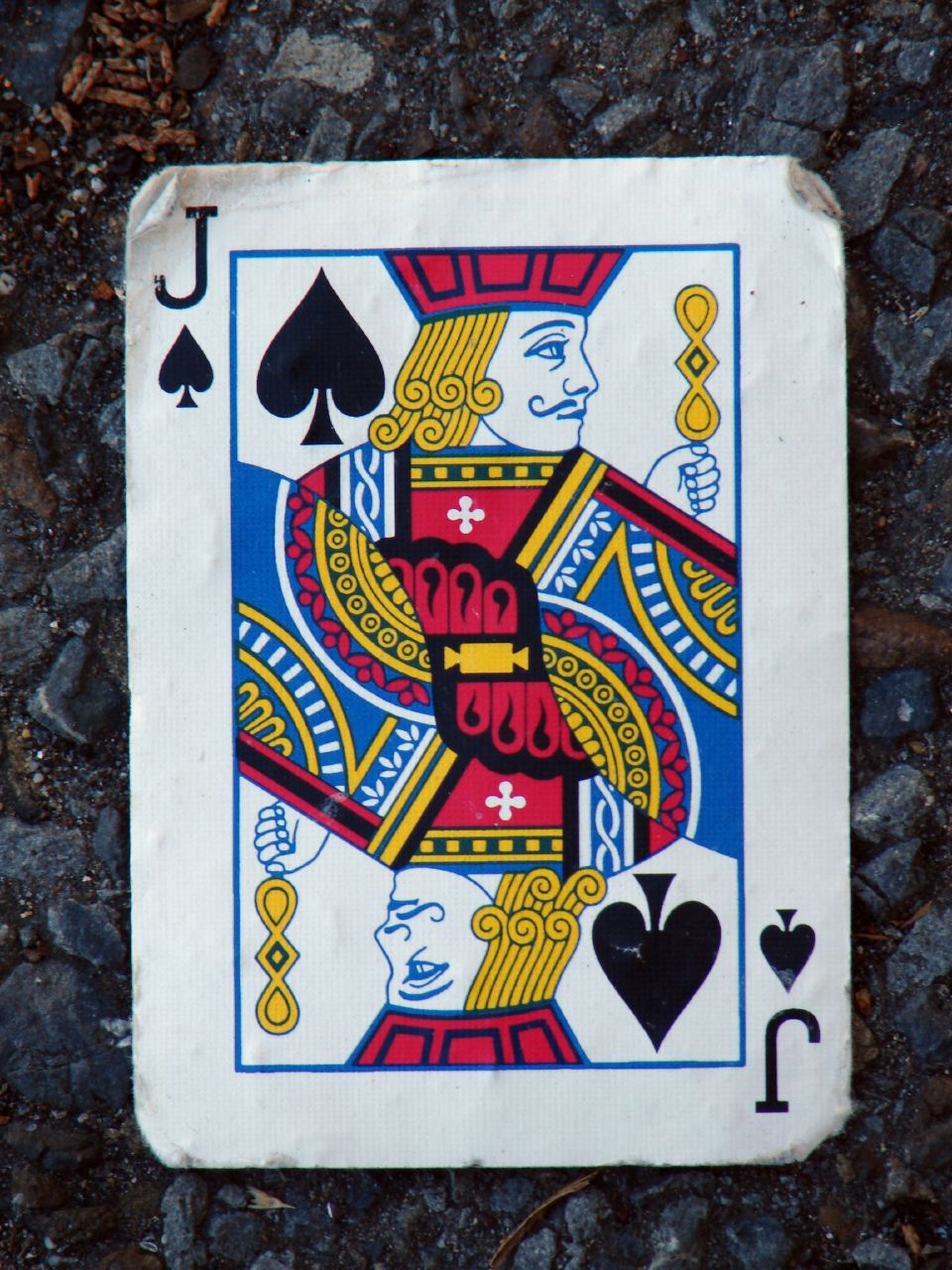In this evocative photograph captured in portrait mode, a well-worn Jack of Spades playing card is prominently displayed face-up on a rugged, uneven surface. The white background of the card starkly contrasts with the weathered, rocky setting that it rests upon, which is filled with numerous crevices and specks of brown debris. The edges of the card are noticeably bent and frayed, indicative of frequent use and handling, a detail that would disqualify it from any professional card game due to the potential for recognition.

The Jack of Spades, depicted with intricate detail, features the traditional mirrored image design. The Jack's eyes are fixed on a gold, teardrop-shaped diamond he holds, adding an air of mystery to the image. He is dressed in a richly decorated coat adorned in red, blue, and white, typical of a standard playing card, possibly from a US standard deck.

In the upper left-hand corner of the image, the texture and imperfections of the rocky surface become more pronounced, with myriad small brown fragments filling the gaps and adding an earthy texture to the composition. The scene's overall effect crafts a narrative of well-used utility and a juxtaposition of human-made and natural elements.